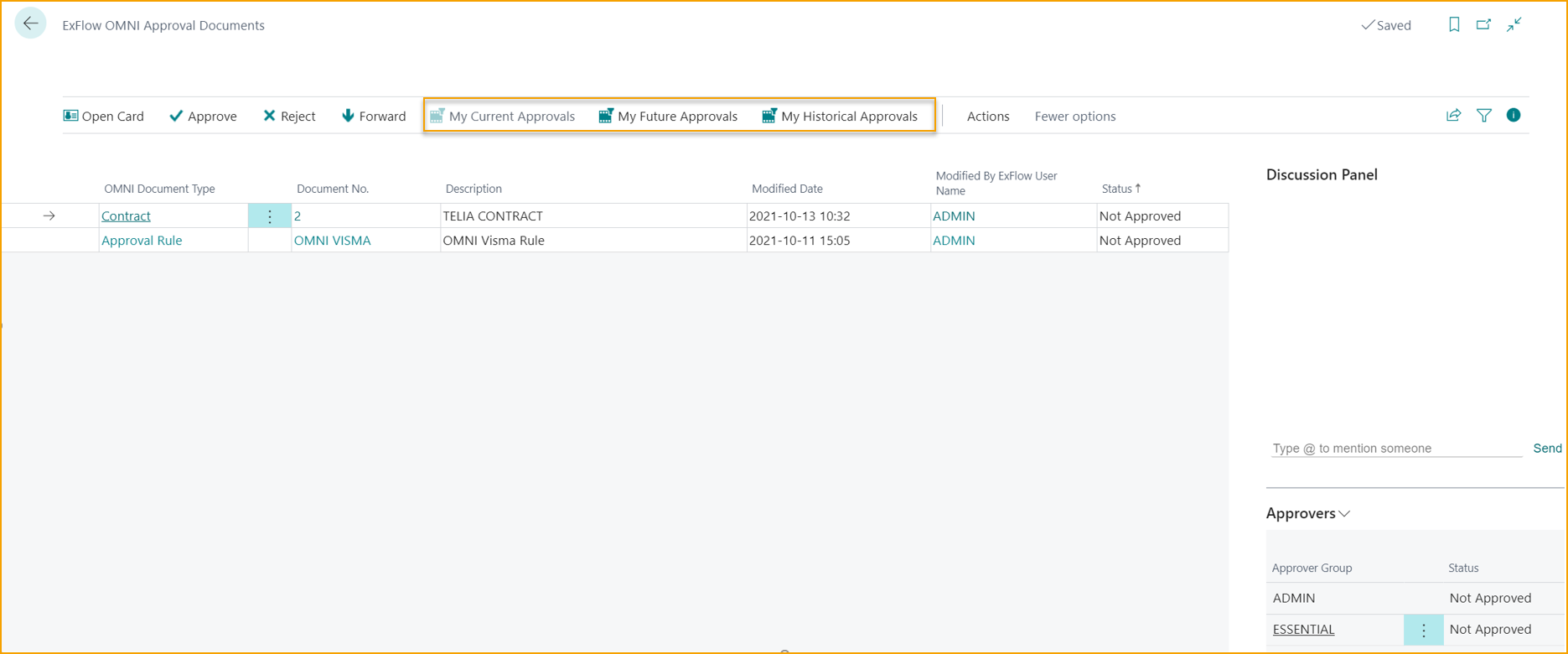A detailed screenshot caption for the given description could be:

---

**Screenshot of a Web-Based Project Tracking Interface**

The screenshot captures a web-based interface centered around project and document approvals, likely part of a management or workflow system. The header includes a left-pointing arrow inside a pale blue circle, with text next to it reading "Xflow Omni Approval Documents."

A comprehensive menu bar below the header offers several options: Open Card, Approve, Reject, Forward, My Current Approvals, My Future Approvals, My Historical Approvals, Actions, and Fewer Options. The sections for My Current, My Future, and My Historical Approvals are highlighted with a gold rectangle, drawing attention to these options.

The main body of the interface is a six-column list designed to track various documents and their statuses. The columns are labeled as follows: Omni Document Type, Document Number, Description, Modified Date, Modified by Xflow Username, and Status. Within this grid, two entries are displayed.

- **Row 1:** 
  - **Omni Document Type:** Contract
  - **Document Number:** 2
  - **Description:** Telia Contract
  - **Modified Date:** 2021-10-13 10:32
  - **Modified by Xflow Username:** Admin
  - **Status:** Not Approved

- **Row 2:** 
  - **Omni Document Type:** Approval Rule
  - **Document Number:** Omni Visma
  - **Description:** Omni Visma Rule
  - **Modified Date:** 2021-10-11 15:05
  - **Modified by Xflow Username:** Admin
  - **Status:** Not Approved

On the right-hand side, a Discussion Panel sidebar is visible, indicating sections for ongoing discussions related to the documents. At the bottom of this panel, a list of Approvers is shown, both labeled as "Admin" and "Essential," with their status marked as Not Approved.

This detailed illustration outlines the key features and layout of the document approval tracking system, highlighting its navigational structure and content organization.